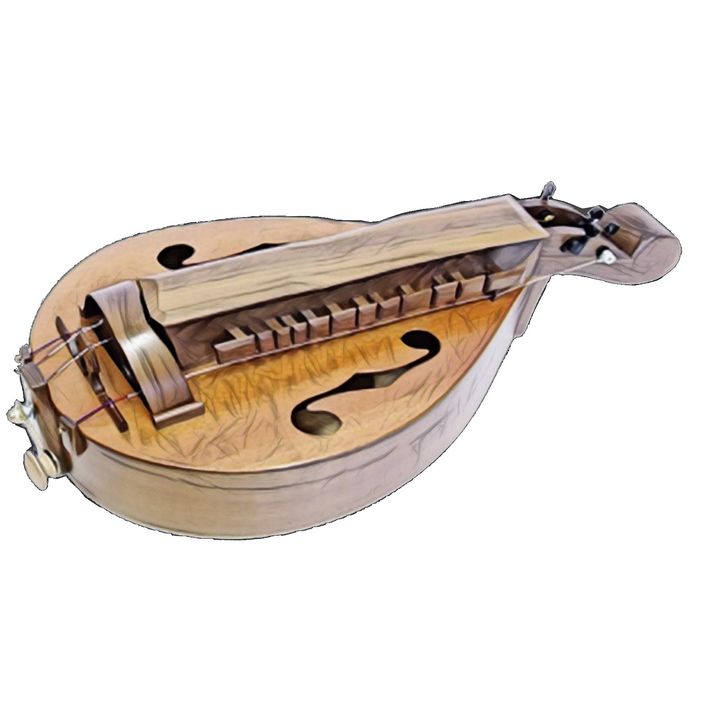This painted image presents a unique wooden string instrument with a teardrop-shaped body that draws a resemblance to both a guitar and a violin. The instrument's body showcases intricate design elements, including a raised board running through the center and two decorative inlay cut-outs on either side. The instrument features a short neck at the top, adorned with a handle that curves thickly at the end, leading to what appears to be tuning areas. The center of the instrument is lined with strings that extend down to knobs situated at the bottom, potentially used for adjusting the tension and tuning. Although some parts of the image appear blurry, the detailing remains evident with noticeable musical note motifs that are reversed and integrated into the design. Additionally, at the bottom left, a few contraptions seem to hold the strings in place, ensuring their stability and functionality. This image seems to be a product photo, albeit slightly unclear, demonstrating a blend of traditional string and potential keyboard elements in a single, elaborate musical device.